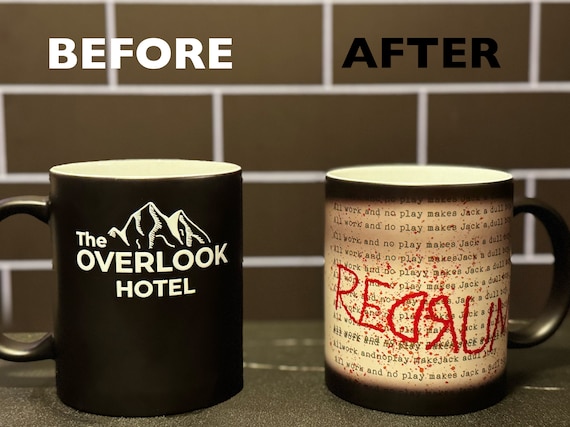The photo features two mugs against a brown brick wall backdrop, partially seen above a light brown table with two noticeable cracks in its surface. The left mug is black with a white interior and bears a white mountain design along with the words "The Overlook Hotel" in white capital letters. Above this, also in white capital letters, it reads "BEFORE." The right mug is light brown with dark brown trim and a matching handle, which faces to the right. This mug has multiple lines of small black text repeating "All Work and No Play Makes Jack a Dull Boy," a reference to the movie The Shining. Across the mug’s center, in large red letters with a bloody design, it says "REDRUM," with the middle "D" and "R" reversed. Underneath "REDRUM," the word "Playmakers" is written. The interior of this mug is also white. The image captures a thematic transition depicted as "Before" and "After" through the designs and inscriptions on the mugs, drawing from iconic elements of The Shining.